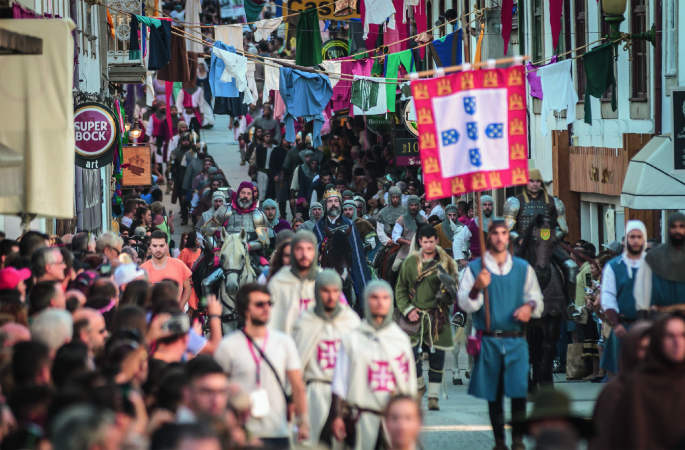In the midst of a bustling city street, adorned with white buildings and clotheslines stretching overhead, a vibrant festival or parade unfolds. The crowded scene is likely set in Europe, featuring throngs of onlookers dressed in modern attire. Central to the spectacle are figures garbed in medieval knight costumes, reminiscent of the Knights Templar. Three men stand prominently, clad in chain mail hoods and white robes adorned with large red crosses, possibly surrounding a kingly figure. To their right, a man dressed like a squire wears a belted blue tunic over a white shirt and hoists a distinctive flag. The flag is square, mounted to a horizontal bar, and features a red border adorned with gold crowns, encircling a white box with blue rectangular shapes inside. The scene is filled with the energy of a lively street parade, with banners, bar signs, and countless onlookers capturing the festive ambiance.